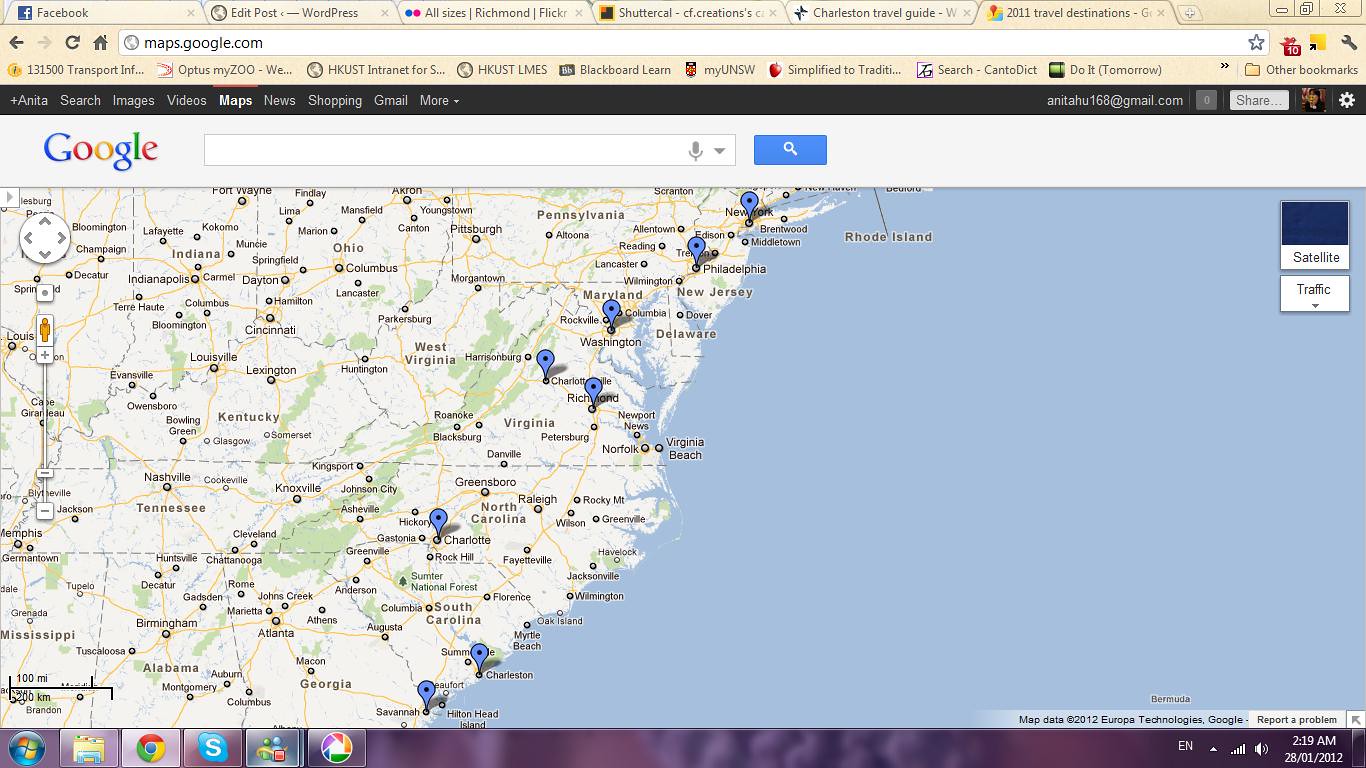This is a detailed, horizontal, rectangular screenshot of a computer screen displaying Google Maps in the main browser tab with the URL maps.google.com visible. The upper left corner shows multiple open tabs including Facebook, Edit Post on WordPress, All Sizes, Richmond Flickr, and Shutter Cow CF Creations, among others.

The map prominently features the East Coast of the United States. It specifically highlights a large body of blue water to the right, representing the Atlantic Ocean. The states visible include Rhode Island, New York, Pennsylvania, Delaware, Maryland, Virginia, West Virginia, Kentucky, Tennessee, North Carolina, South Carolina, Georgia, Alabama, Mississippi, and parts of Indiana and Ohio. Cities such as New York, Philadelphia, Washington, Richmond, Charlottesville, Charlotte, Charleston, Savannah, Huntington, Lexington, Nashville, Chattanooga, and Indianapolis are marked with dark blue pins featuring black dots in the center.

The Google logo is displayed above the map in its traditional color scheme: blue 'G', red 'o', yellow 'o', blue 'g', green 'l', and red 'e'. Above the map is an empty search bar. The bottom edge of the map features a purple horizontal line with various icons, including a folder, and the system time displayed in white font at the bottom right corner. The map details show regions extending from Pennsylvania in the north to Georgia in the south.